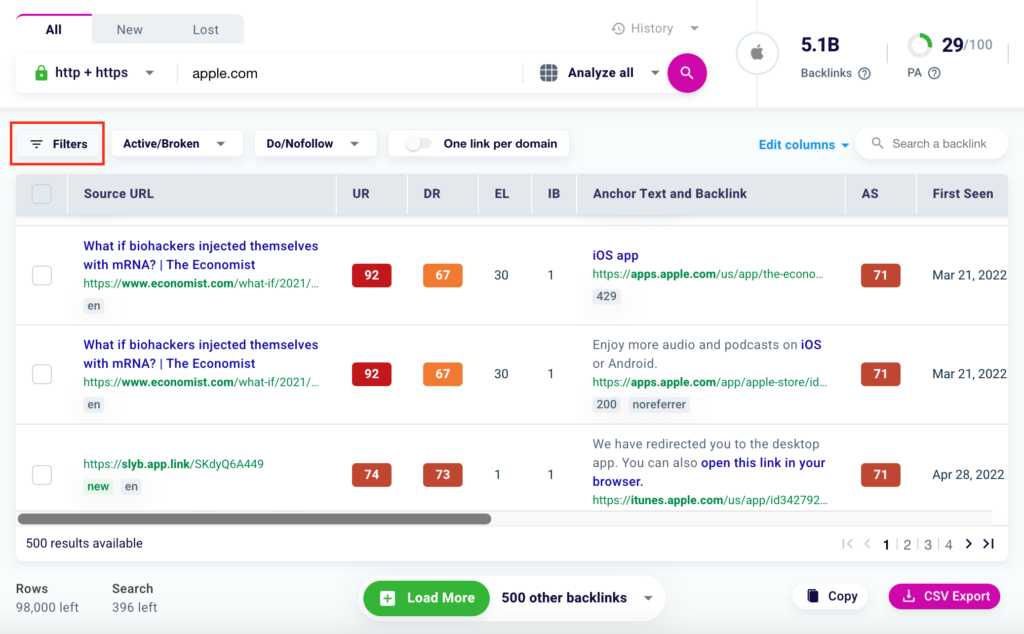This is a detailed screenshot of a web page, presumably an SEO or backlink analysis tool. 

At the top, the toolbar contains several tabs and options labeled: "All," "New," "Lost," "HTTP plus HTTPS," "apple.com," "History," and "Analyze All." Additionally, it displays metrics like "5.1b Backlinks" and "29/100 PA." This section is highlighted with a red rectangle.

Below the toolbar, various filter and customization options are available: "Active/Broken," "Do/Nofollow," "One Link per Domain," "Edit Columns," and "Search a Backlink."

The table beneath these options includes the following columns: "Source URL," "UR," "DR," "EL," "IB," "Anchor Text and Backlink," "AS," and "First Seen."

Highlighted rows within the table include details such as:

1. **First Row:**
   - **Anchor Text and Backlink:** "What if biohackers injected themselves with mRNA, The Economist?"
   - **Metrics:** "92, 67, 30, 1"
   - **Additional Information:** "iOS app, 71, March 21st, 2022"

2. **Second Row:**
   - **Anchor Text and Backlink:** "What if biohackers injected themselves with mRNA, The Economist?"
   - **Metrics:** Same values as above: "92, 67, 30, 1"
   - **Additional Information:** "Enjoy more audio and podcasts on iOS or Android, 71, March 21st, 2022"

3. **Third Row:**
   - **URL:** "https://slyb.app.link/SKDYQ6A449"
   - **Metrics:** "74, 73, 1, 1"
   - **Additional Information:** "We have directed you to the desktop app. You can also open this link in your browser. 71, April 28, 2022"

At the bottom of the page, there are options to navigate and manage the data, including "500 results available," "Rows 98,000 left," "Search 396 left," "Load More," "500 Other Backlinks," "Copy," and "CSV Export."

Overall, this screenshot provides an in-depth view of the tool's capabilities for analyzing and managing backlinks, complete with filtering and exporting functionalities.